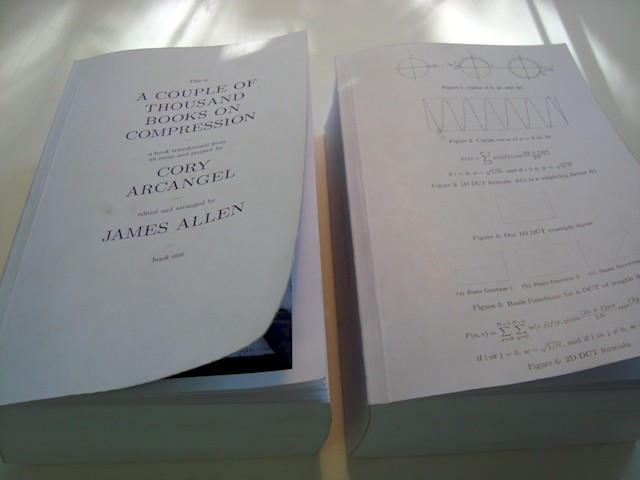This image features a photograph of two thick, potentially two-inch paperback books, laying side by side on a table, both resting on a green stand. The book on the left shows the front cover, which is white with dark purple lettering, stating "A Couple of Thousand Books on Compression" by Cory Arcangel and edited and arranged by James Allen. The book on the right appears to be opened to an inner page filled with diagrams. At the top of the right book's page are circular diagrams connected by lines, with a series of up-and-down lines underneath, resembling a radio frequency graph. Below these diagrams, dark print extends towards the bottom of the page, though it is too small to read clearly in the image.